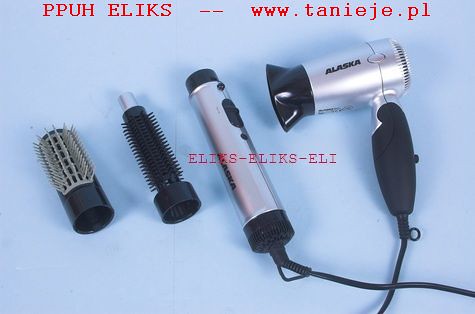This rectangular image, wider than it is tall, features an advertisement for hair styling tools against a light periwinkle blue background. At the top, in bold red letters, is the text "P-P-U-H E-L-I-K-S -- www.tanieje.pl". In the center, also in red letters, is "E-L-I-K-S - E-L-I-K-S - E-L-I".

The main subjects of the image are a silver and black hairdryer and a curling iron with interchangeable attachments. The hairdryer, positioned on the right, is compact and has a black handle with the word "Alaska" displayed prominently in the center. A cord extends from the bottom of this hairdryer.

To the left, the curling iron is distinguishable by its cylindrical silver body with black accents and buttons, and a similar "Alaska" branding. Next to the curling iron are two attachments—a round brush with black bristles and a regular brush with white-gray bristles, both designed to snap onto the curling iron for versatile styling.

The clarity and organization of the image highlight each hair accessory's purpose and design, making it easy to understand the utility of the products being advertised.